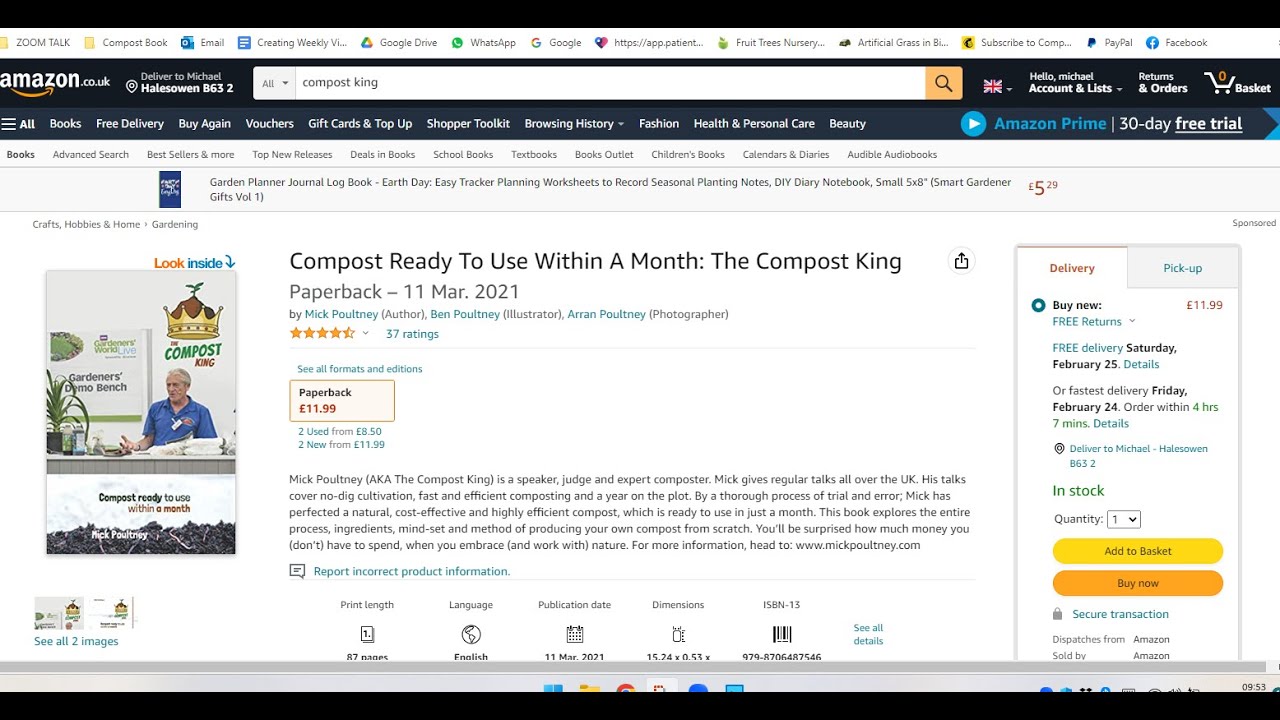**Caption:**

Screenshot of the UK version of Amazon's product page featuring the paperback book "Compost King" by Mike Pulteney, priced at €11.99. The user, logged in as Michael at Hallazween B63, is considering adding the book to his basket. Currently, his basket is empty, but he has the option to add the book for delivery or pickup, with free returns available. 

"Compost King" has garnered 37 ratings, boasting an impressive 4.5 out of 5 stars. It is in stock and can be delivered by Saturday, the 25th if ordered within the next four hours. An Amazon Prime 30-day free trial advertisement is displayed beneath the product details. 

The cover of the book features the title "Compost King" in green, with an image of Mike Pulteney at a press conference, wearing a blue polo shirt with a red emblem and a crown graphic above his head. To the left of him is a plant. The description highlights Pulteney's credentials as a speaker, judge, and expert composter who regularly conducts talks in the UK. Additional book details such as print length, language, publication date, dimensions, and the ISBN number are listed below the description.